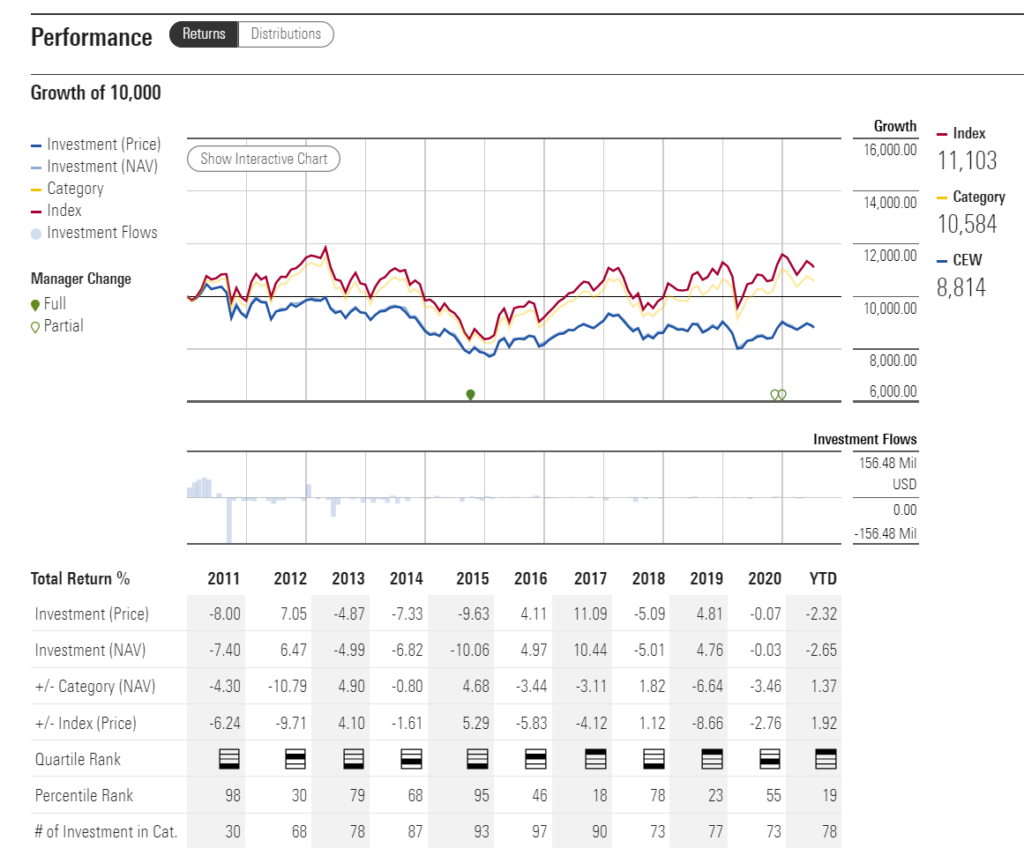This image is a detailed investment performance chart. In the upper left-hand corner, it is labeled "Performance" with sections for "Returns" in black and "Distributions" in white. The chart prominently features the growth of a $10,000 investment over time. Key elements of the chart include:

- **Color-coded Legend**: 
  - Investment Prices (Blue)
  - Investment NAV (Gray)
  - Category (Yellow)
  - Index (Red)
  - Investment Flows represented by light blue dots

- **Graph Dynamics**:
  - The chart showcases various color-coded lines indicating different aspects of the investment.
  - Initially, the graph is stable, then dips down, followed by an upward trend. This pattern repeats with another dip and a subsequent increase.
  
- **Manager Change Indicators**:
  - "Full" manager changes are marked in green, while "Partial" manager changes are marked with uncolored icons.
  
- **Growth Column**: 
  - Provides numerical values showing growth over time.
  
- **Additional Graph**:
  - Below the main chart is a light-colored bar graph depicting investment flows, which shows higher activity initially that slows down over time.
  
- **Total Return Percentages**:
  - At the bottom, total return percentages are displayed for each year from 2011 to 2020, including a year-to-date figure.

- **Interactive Element**:
  - A note at the top indicates the availability of an interactive chart.

The overall visualization offers a comprehensive look at the investment's performance, with detailed data aiming to provide a clear historical perspective.